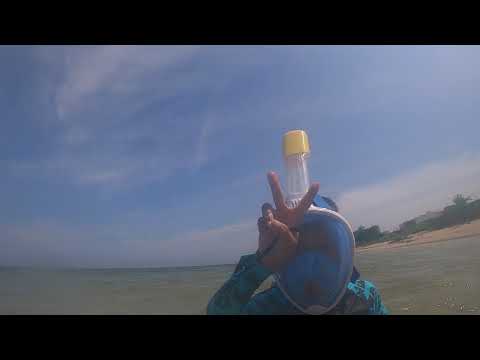The image depicts a person waist-deep in greenish water, wearing a blue snorkeling outfit complete with a large, opaque, blue face mask covering their entire face. A white cylindrical snorkel attachment with a yellow cap extends from the top of the mask. The person is gesturing a peace sign with their right hand, which is positioned in front of them with the palm facing outward. Only their head and shoulders are visible. The background features a serene blue sky with a few clouds, a strip of sandy shore, and some trees on the right side of the frame. The overall atmosphere suggests that the person is engaged in a water-based activity, possibly snorkeling or collecting samples, while enjoying a tranquil natural setting.